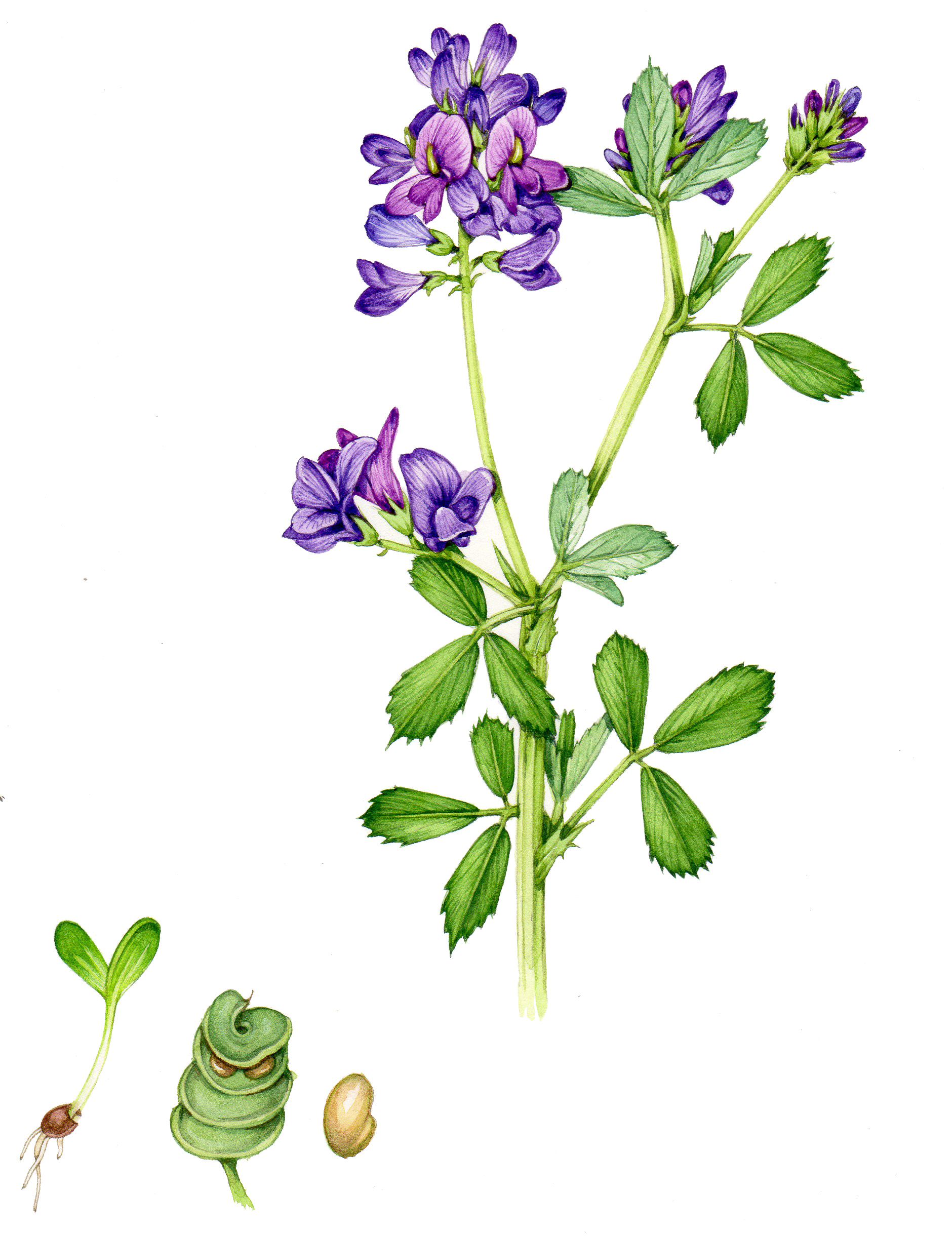This image shows a detailed painting or digital artwork of a flowering plant set against a white background. The main focus is a plant with a green stem that bifurcates into two branches. The plant features numerous green leaves, each cluster comprising three pointed leaves. The plant is adorned with delicate purple flowers. One branch at the lower part has three blooms, while the higher branch boasts five blooms, with additional buds yet to open. The right branch also has several unopened buds. In the lower left-hand corner of the image, there are three smaller diagrams: one shows a newly sprouted seedling with roots, the second depicts a spiral form encasing a seed, possibly illustrating the plant's seed development process, and the third shows a brown oval seed. The artwork is noted for its clean and unique design, with the recurring elements of green leaves and purple flowers providing a cohesive visual theme.